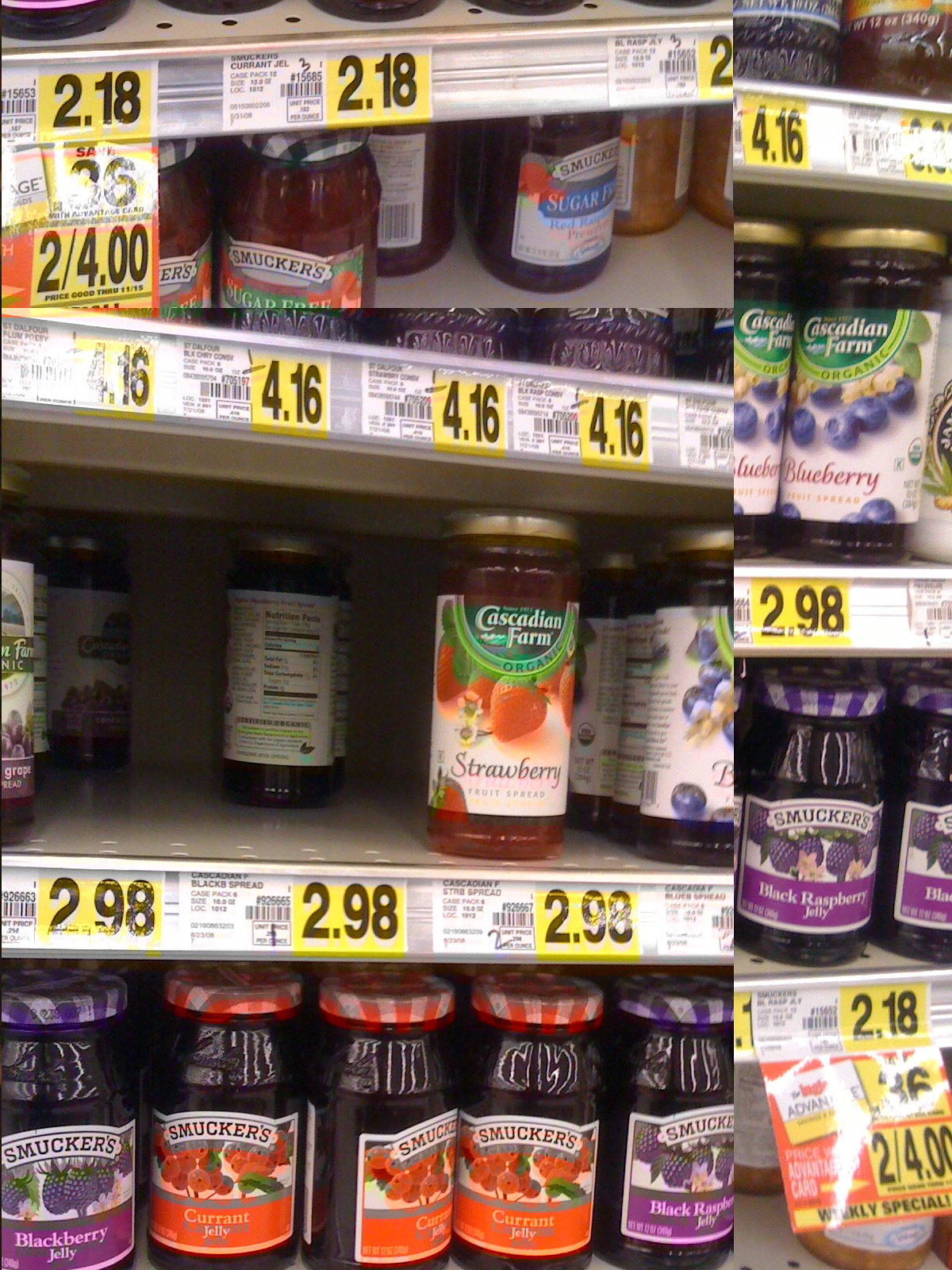The image depicts a supermarket shelf stocked with various jams and jellies. The layout features two photos combined side by side, forming a single vertical composition that's longer on the vertical axis. The right 30% of the image is a close-up of items on the store shelf, highlighting the details of the products and their prices. 

On both sides of the image, the shelves display an assortment of jams and jellies, prominently featuring two brands: Cascadian Farm and Smucker's. At the bottom row on the left side, rows of Smucker's jars are arranged, displaying flavors such as currant, blackberry, strawberry, and grape. Some of these Smucker's products, including the blackberry and raspberry jellies, are on a weekly special offer of two for $4. Regular prices for Smucker's jams are also visible, with some jars priced at $2.18.

Directly above the Smucker's items on the left, there are jars from Cascadian Farm, including flavors like organic blueberry, blackberry, and strawberry. The price for Cascadian Farm's organic blueberry jelly is $2.98, as indicated on a yellow price tag. Notably, the Cascadian Farm blackberry spread appears to be popular, with only two or three bottles remaining.

Overall, the intricate arrangement of jars and clearly marked prices, with yellow and black tags, provides a detailed and inviting display of the jam selection available at the store.